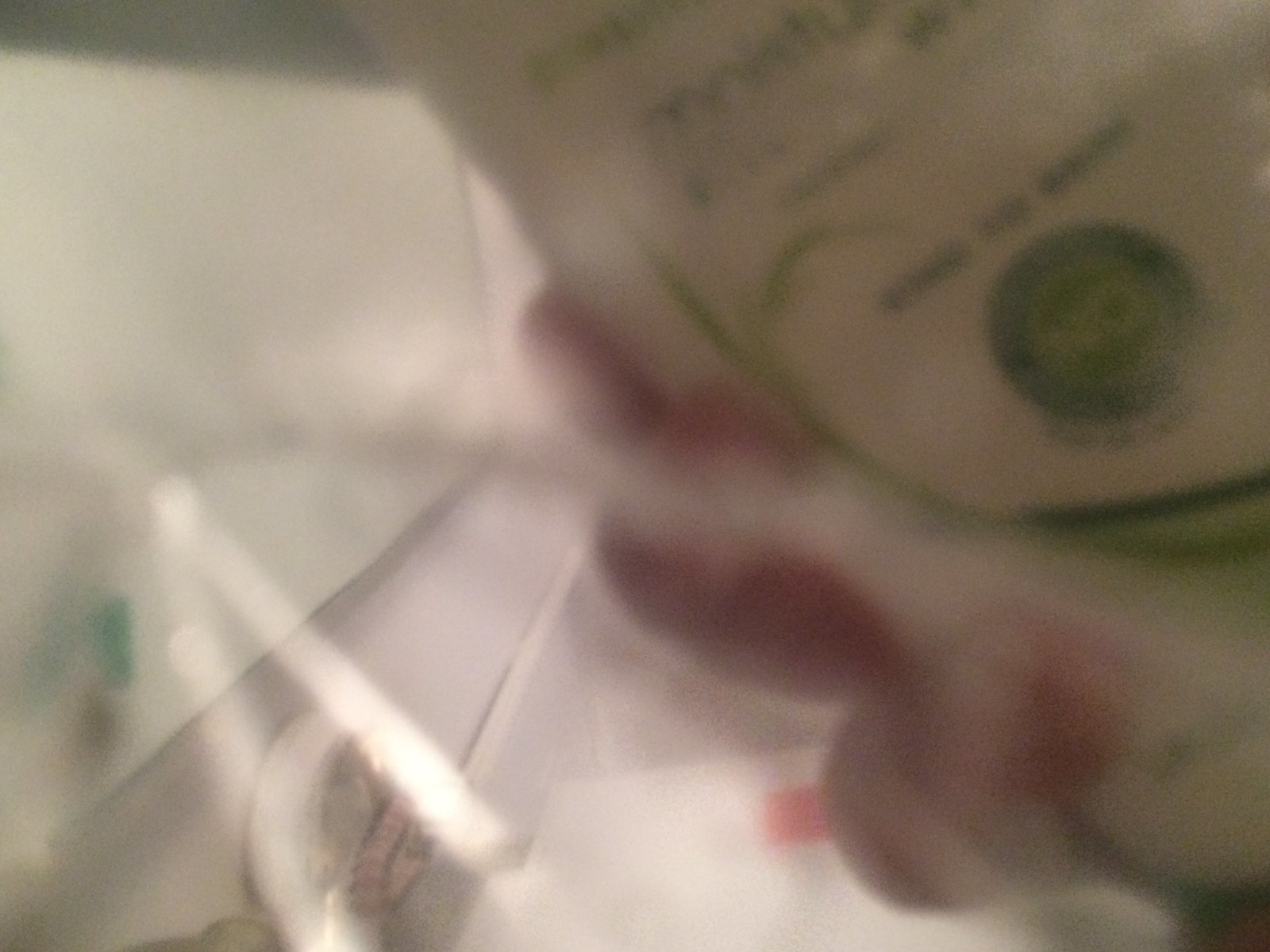The photograph is extremely blurry and difficult to decipher, resembling an accidental close-up shot. Predominantly, it appears to capture a person's hand entering from the right side of the image, holding a white and greenish bag of food, which takes up nearly half of the picture and is angled to display its front. The fingers gripping the bag are near the lower center. On the left side, there are various containers and reflections suggesting a possible bathroom setting. Additional details include an upside-down bottle with a visible "O" and "N" and some green and pink hues adding to the confusion of the image. The background is lit, though the entire photo lacks legible text and discernible focal points.